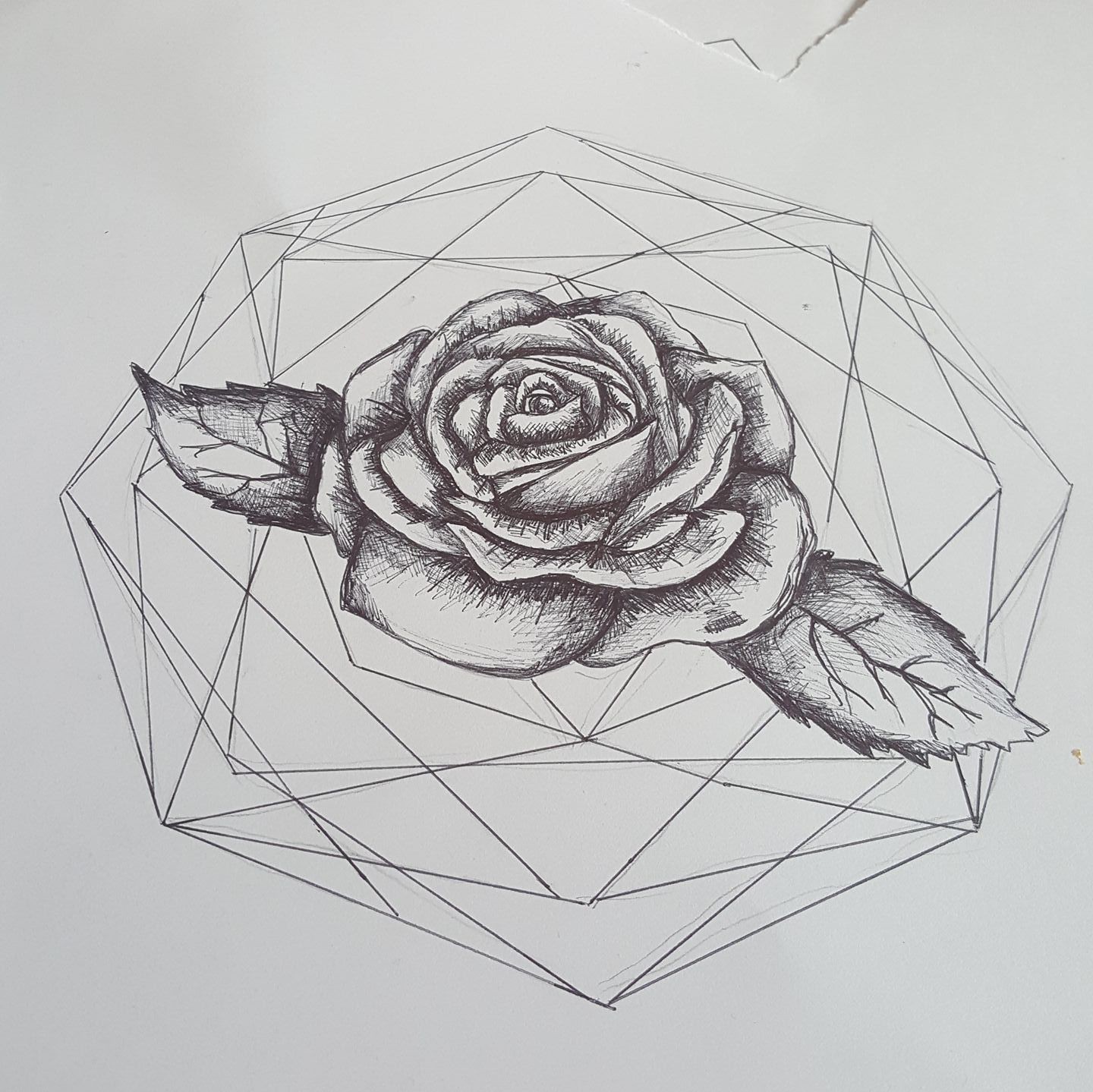This intricate drawing, rendered on white paper with pen or pencil, combines the precision of geometric shapes and lines with the organic beauty of a rose. The artwork features black geometric figures and intersecting lines that frame and guide the viewer's attention to the center, where a meticulously shaded rose blooms prominently. The rose, with numerous visible petals, showcases detailed shading that adds depth and realism to each delicate petal and the adjoining leaves. The leaves, positioned on either side of the rose, exhibit serrated edges and pronounced veins, further enhancing the botanical accuracy and texture of the piece. The interplay between the stark, structured geometry and the soft, natural elements of the rose creates a harmonious and captivating visual experience.